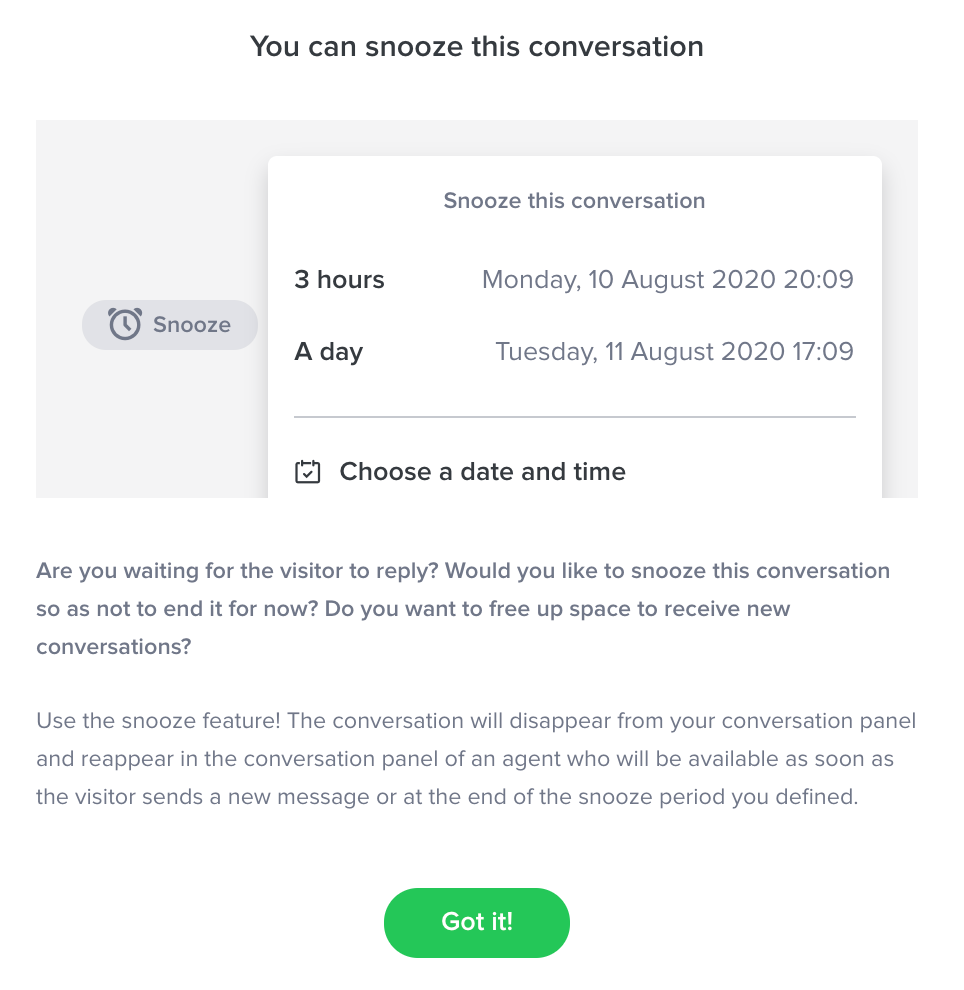The image features a user interface for snoozing a conversation. At the top, in bold black font, it reads "You can snooze this conversation." Below this, a section shows an icon of an alarm clock with clock hands and two dots, accompanied by the word "snooze." To the right, it states "Snooze this conversation," followed by the bold text "Three hours" in black. Next to this, it displays "Monday, 10th August 2020, 20.09." 

Below this first section is another line with the day "Tuesday, 11th August 2020, 17.09." Further down, a rectangle with the label "Choose a date and time" in dark black text can be seen. The interface asks, "Are you willing for the visitor to reply? Would you like to snooze this conversation so as not to end it for now? Do you want to free up space to receive new conversations?"

It then suggests using the snooze feature, stating, "The conversation will disappear from your conversation panel and reappear in the conversation panel of an agent who will be available as soon as the visitor sends a new message or at the end of the snooze period you defined." At the bottom of the image, a green circle contains the text "Got it."